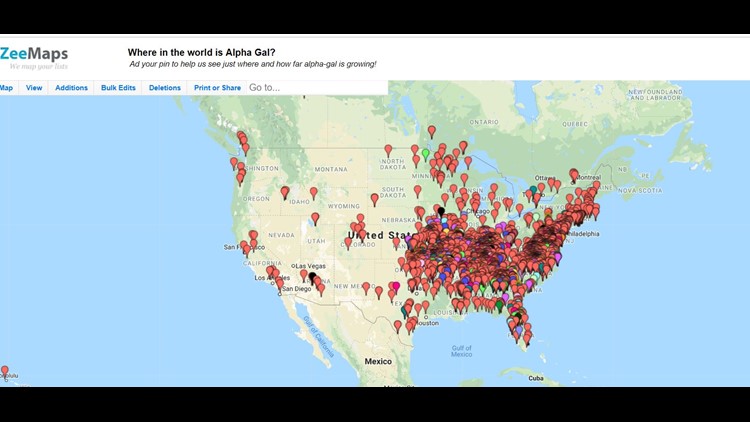This image depicts a web page featuring a detailed map. The top of the page is bordered by a black strip, below which is the heading "Zmaps" with the tagline "We map your lists." The central text reads, "Where in the world is AlphaGal? Add your pin to help us see just where and how far AlphaGal is growing." The web page includes a variety of tabs labeled "Map," "View," "Editions," "Bulk Edits," "Deletions," and "Print or Share." There is also a "Go-To" section that functions as a text box for navigation.

The main focus of the image is the map of the United States, displaying numerous colored dots representing different locations. The majority of these dots are red and are densely clustered in the Midwest, South, and the Eastern United States. Scattered clusters are visible, with fewer pins in regions like California and Colorado. While the predominant color of the pins is red, there are occasional green and purple pins interspersed throughout. The map also includes a blue section depicting bodies of water for added geographical context. At the bottom of the image, another black bar runs across, reinforcing the webpage-like appearance of the visual.